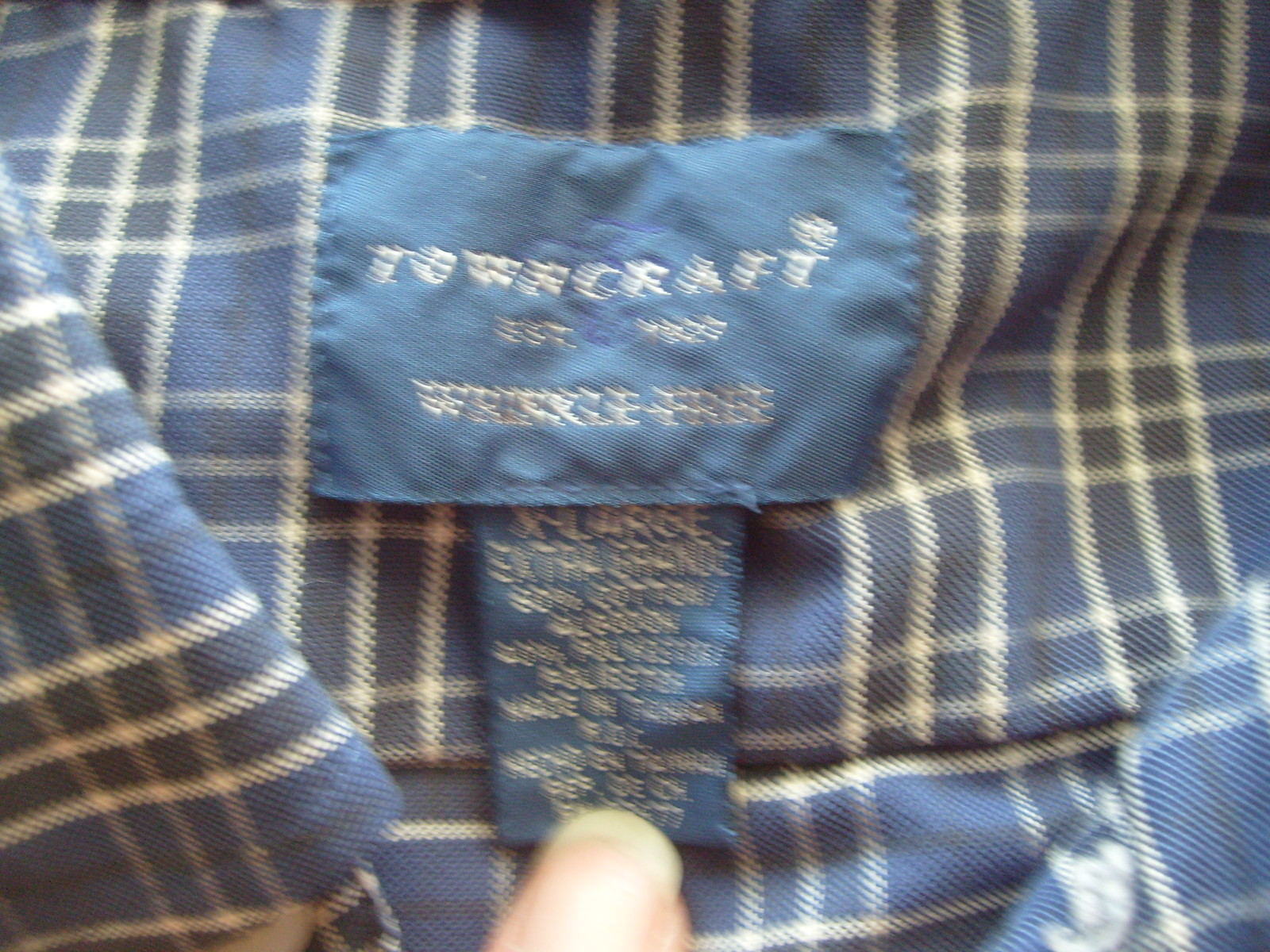The image showcases the interior label of a piece of clothing, likely a button-up shirt or blazer, crafted from a blue and white checkered plaid fabric. The label, positioned centrally in the photograph, displays the brand "Towncraft." Although the year printed below the brand is blurry and hard to decipher, it appears to be around 1927. Further down, the words "wrinkle-free" are clearly visible. The label itself is blue, with white stitching that stands out prominently. Beneath this, an additional tag indicates the size as Extra Large and details the fabric composition as 60% cotton and 40% polyester, made in Taiwan. To stabilize the label for the photograph, a fingernail is visible at the bottom center of the image, suggesting the owner is holding it in place.